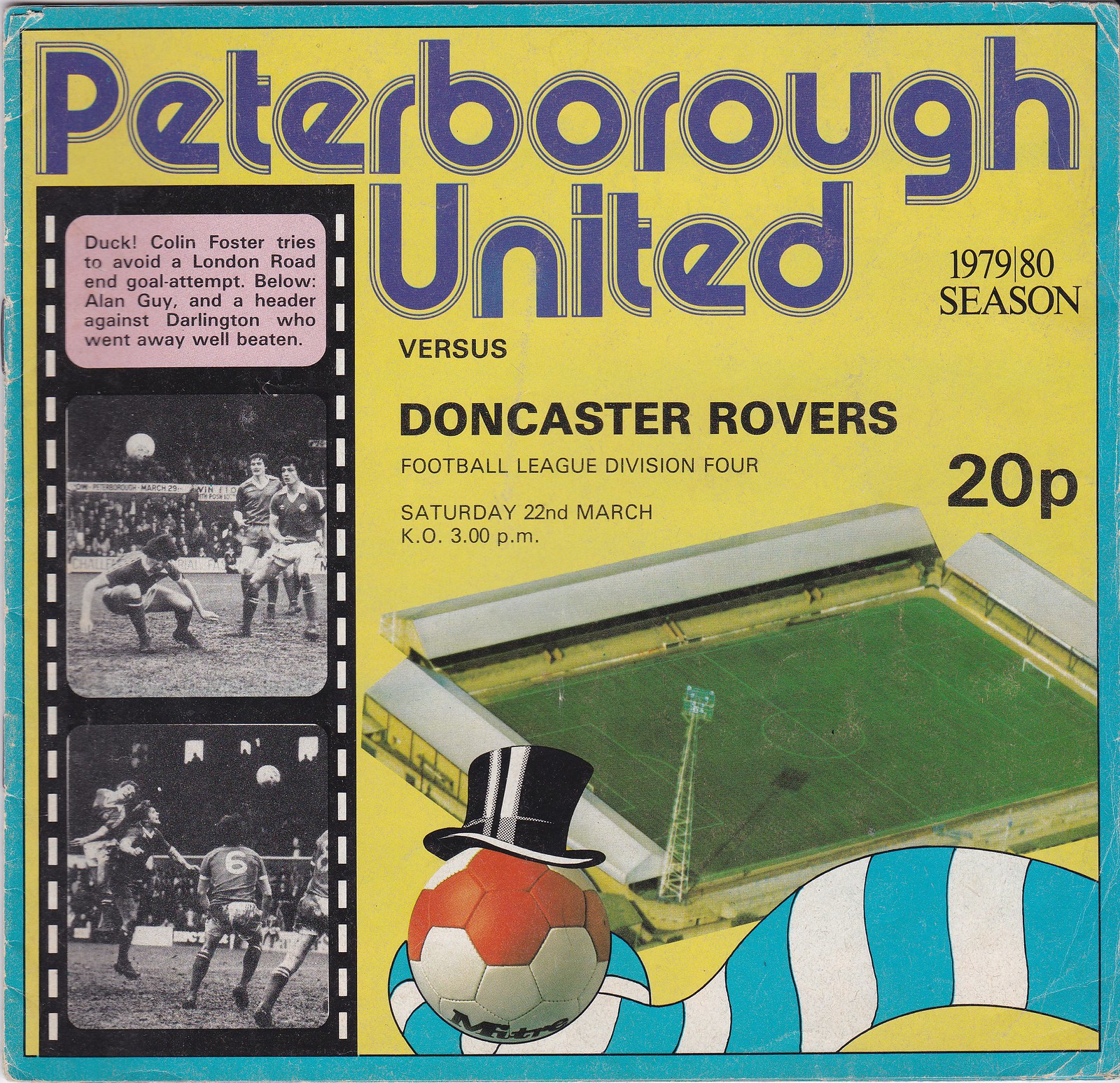This advertisement from the 1979-1980 football season captures the lively spirit of a much-anticipated match between Peterborough United and Doncaster Rovers in Football League Division 4. The backdrop of the ad features a vibrant yellow with a contrasting blue border, drawing attention to the central imagery and text. 

In the bottom center of the ad, a whimsical graphic of a red and white soccer ball donning a black top hat stands out. Behind it, there’s an aerial view of the stadium where the match is set to take place, giving a sense of locality and excitement.

On the left side, a vertical film reel displays two dynamic scenes from soccer matches. The top photo is captioned, "Duck, Colin Foster tries to avoid a London Road end goal attempt," depicting a tense moment in gameplay. The second photo underneath reads, "Below, Alan Guy and a header against Darlington who went away well beaten," capturing a victorious instance.

The top of the advertisement prominently features text announcing the event: "Peterborough United" and "Versus" in grey font, and "Doncaster Rovers" in bold black font. Additional details inform fans that it is a Football League Division 4 match scheduled for Saturday, the 22nd of March, with kickoff at 3 PM. Positioned to the far right, the number "20p" suggests that admission to this thrilling match is priced at 20 pence, making it an accessible event for fans.